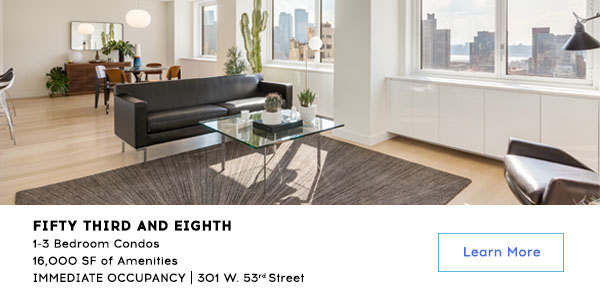This image is a screenshot of a rental apartment located in a high-rise condominium in a bustling metropolitan area. The photo captures a sophisticated living room with pale wooden floors adorned by a gray area rug. The modern furnishings include a sleek black rectangular sofa and a minimalist glass coffee table, which showcases two potted plants in white planters. Beyond the living area, a cozy dining space is visible, featuring a wooden table with three chairs, illuminated by an elegant white oval hanging lamp. A stylish brown wooden sideboard with a mirror above it completes the dining area decor. A striking large cactus plant stands prominently in the corner by the window, adding a touch of greenery to the urban setting.

Outside the expansive windows, a panoramic cityscape unfolds, hinting at the apartment's prime location in a vibrant city. The text overlay at the bottom of the image reads: "53rd and 8th, one to three bedroom condos, 16,000 square feet of amenities, immediate occupancy, 301 West 53rd Street." To the right, a call-to-action button in blue text edged in a lighter blue invites viewers to "Learn More."

This detailed description highlights the apartment's elegant design, strategic location, and the extensive amenities offered, perfect for prospective tenants seeking upscale urban living.